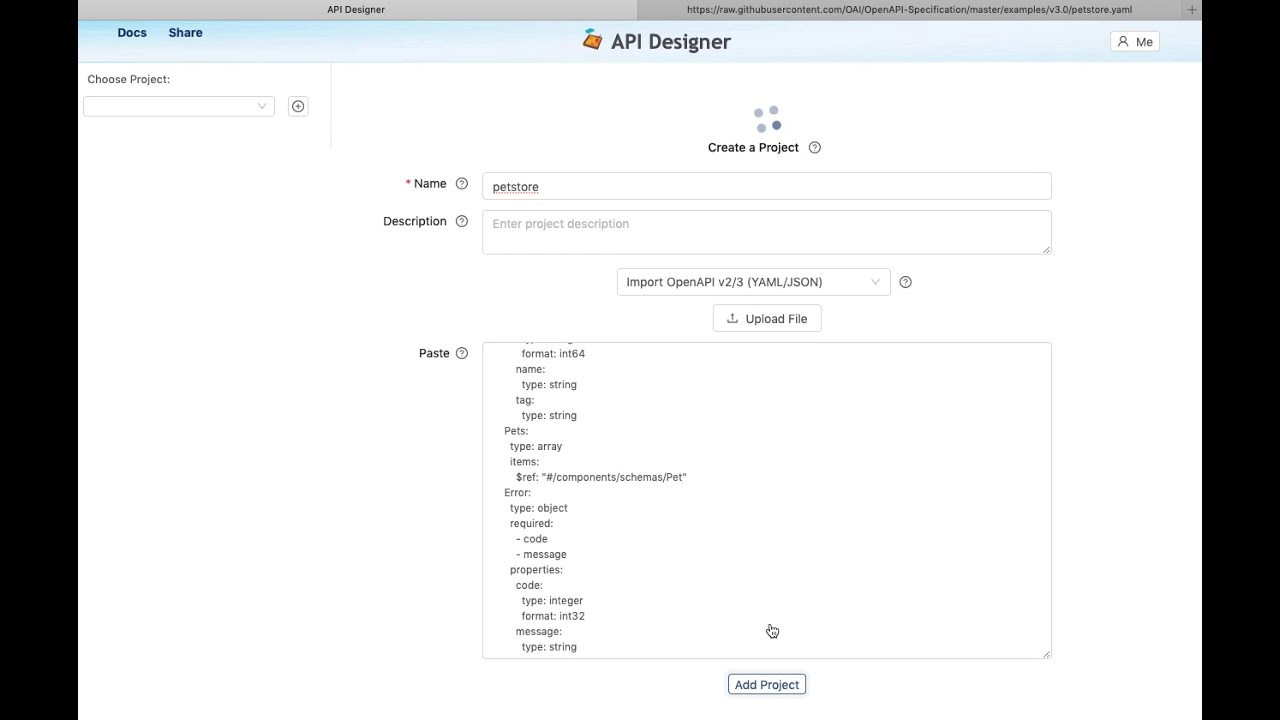The image is a wide rectangular screenshot of a project creation interface on a website. Black vertical bars frame the left and right sides of the image. At the top, a gray bar transitions from light to dark gray and displays "API Designer" on the left and a website link on the right. Below this bar, a light blue gradient rectangle features "Docs Share" in blue font on the left, "API Designer" in gray font in the middle, and a white rectangle labeled "Me" with an animated figure on the right.

The main body of the screen is white, with the top section reading "Create a Project" in black font. Beneath this, there are designated fields for "Name" and "Description," as well as a larger section titled "Paste" for inserting code or an Open API. The interface also includes options such as "Import Open API," "Upload File," and a final button that says "Add Project." The design is clean and user-friendly, emphasizing the name and description fields central to the project's creation.